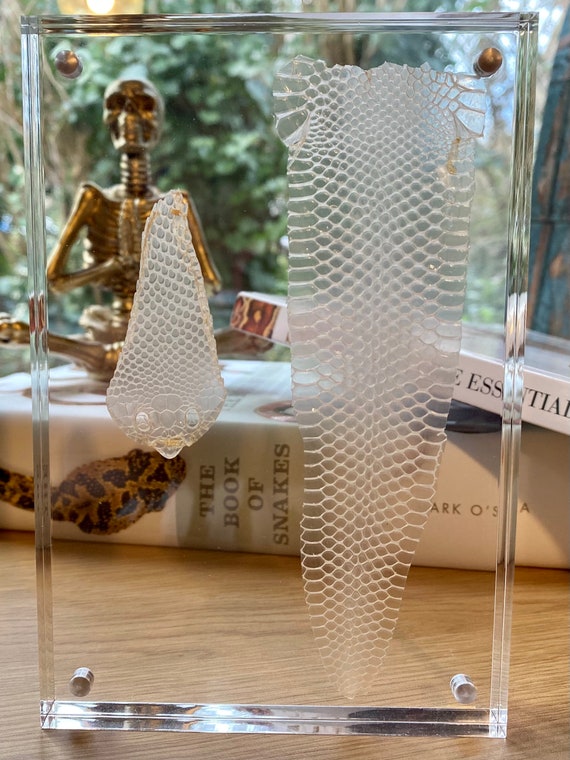In this detailed image, we see a transparent, glass display case positioned directly in front of us. Inside the case, the severed skin of a snake is meticulously arranged, with the snake’s head placed on the left side and the body on the right. The snake scales are almost transparent, revealing intricate details of their former life. The glass case itself is tall and slender, featuring small openings at each corner for accessibility.

Behind this case, there are two books. One book, lying on its side, prominently features the title "The Book of Snakes" along with an illustration of a snake. A larger book rests on a table with the word "essential" visible on its cover. Atop these books sits a golden skeleton figurine in a meditative pose, adding an intriguing element to the scene. In the background, there's an open window, offering a view of the outdoors and completing the composition of this captivating display.